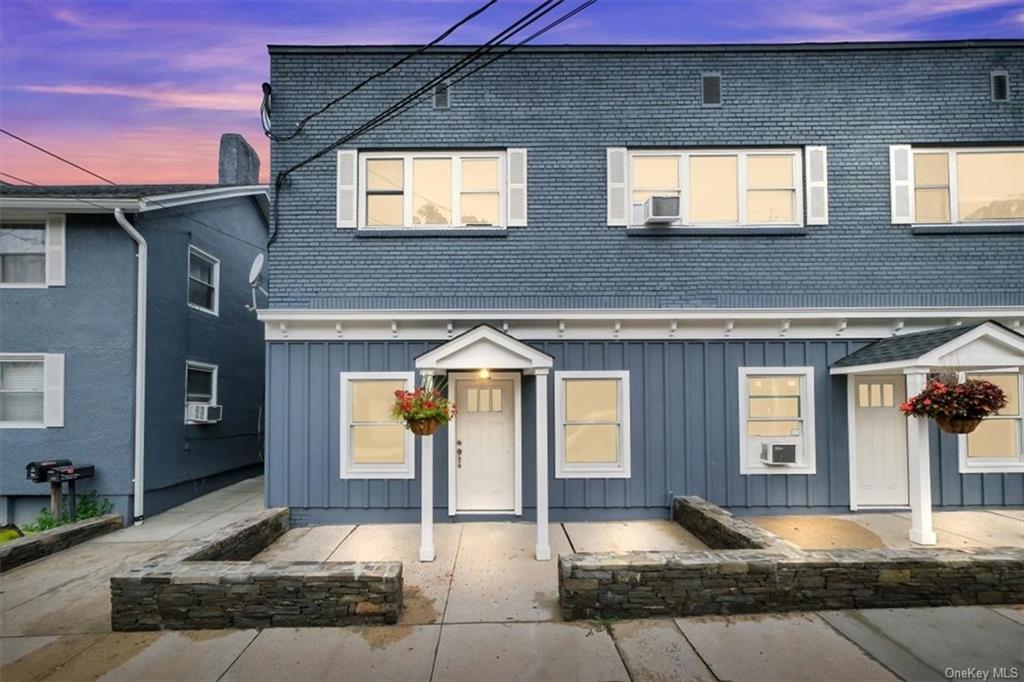This image captures a two-story, multi-unit residential structure that appears to have been converted from an older commercial warehouse or business, now remodeled into living spaces. The building exhibits a mix of historic and contemporary design elements: the upper story retains an older aesthetic with blue brick and newly installed windows, complete with window air conditioners, while the lower level features vertical siding. The flat-roofed front facade includes visible vents, highlighting its past industrial function. There are charming entryways with small roofs supported by square pillars, adorned with hanging plants and bordered by low brick platforms and a paver-fenced area separating it from the street. The scene is set at sunset, with a dark blue sky accented by pink clouds. An alleyway divides the main building from a neighboring, more modern structure.